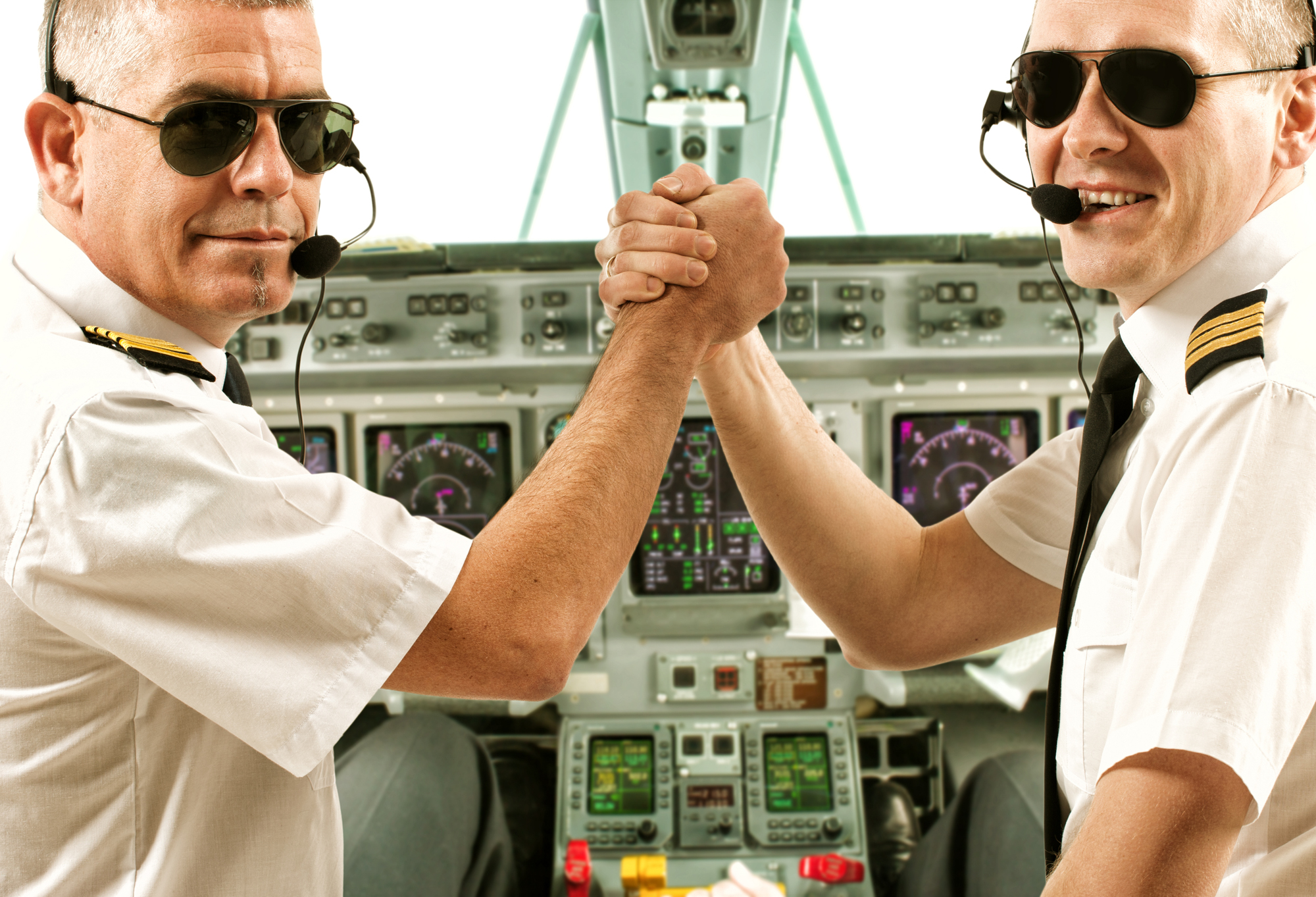The image is a color photograph capturing two airplane pilots seated in the cockpit. The scene is set in a landscape orientation, showing them turned slightly at their shoulders to look back and smile at the camera. Clad in white, short-sleeved shirts with black ties, they sport black sunglasses and headsets with microphones near their mouths. The shoulder epaulettes, adorned with black and gold stripes, signify their rank. The pilots, seated side by side, have their right hands raised and clasped together in a celebratory gesture. The cockpit in the background is filled with a complex array of dials, buttons, and radar screens, with light streaming through the clear windshield, highlighting the detailed control panel in gray hues. The image embodies a sense of camaraderie and professionalism amidst the high-tech environment of the aircraft controls.